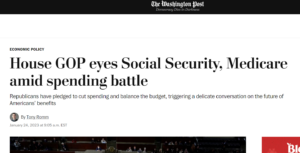This is an online screenshot of the top portion of a Washington Post article. The Washington Post logo is displayed prominently at the top in white calligraphy on a black rectangular background. Directly below, the article falls under the "Economic Policy" section. The headline, "House GOP Eyes Social Security, Medicare Amid Spending Battle," is presented in bold print. It is followed by a subheadline that reads, "Republicans have pledged to cut spending and balance the budget, triggering a delicate conversation on the future of Americans' benefits." The byline indicates that the article is authored by Terry Roman, although the date is blurred and unreadable. The image is zoomed in on the article, cutting off the surrounding content, with a fragment of an adjacent red-highlighted article visible along the edge. Below the text, there appears to be an image which is partially visible.